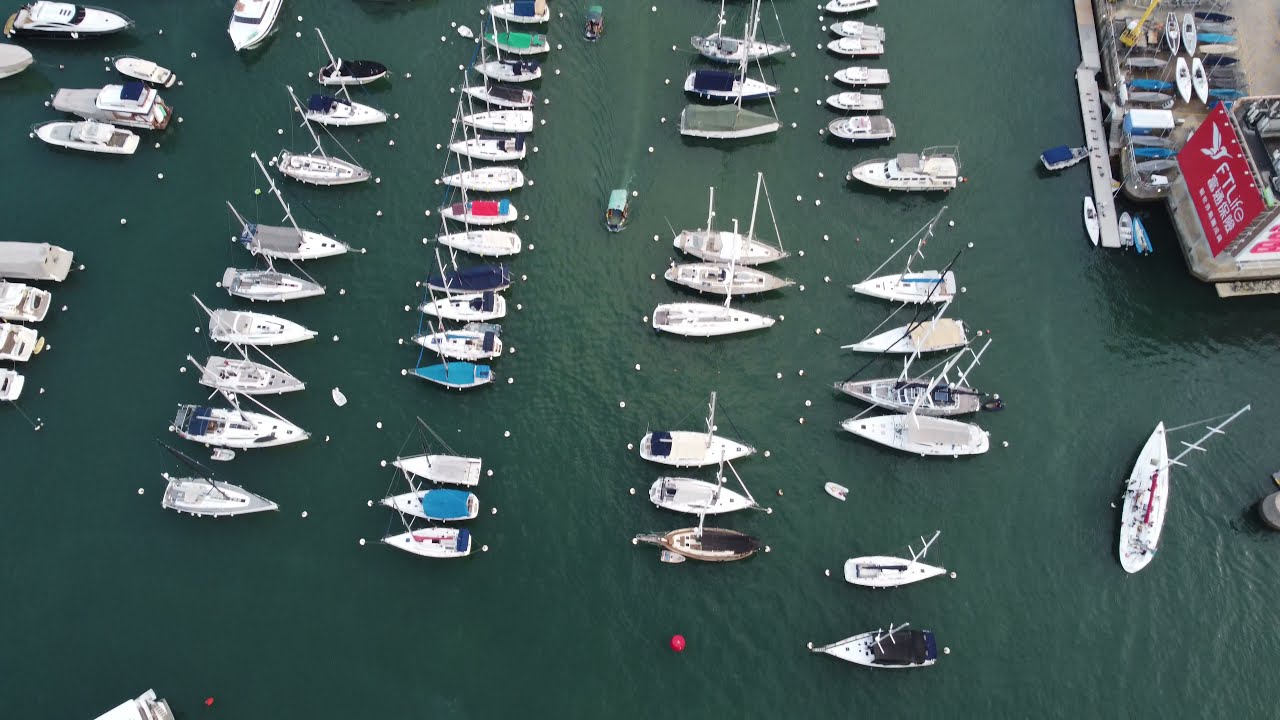The image is an aerial, color photograph taken from a drone, showcasing a marina with a fleet of sailboats organized in five neat, vertical rows. Located in the top right corner is a wooden dock, featuring racks of kayaks and canoes, identified by a prominent red banner reading "FT Life" and a brand logo. The marina waters, a dark greenish-blue hue, reflect the slightly overcast sky. A small, covered vessel is seen patrolling between the moored sailboats, which are anchored with buoys and properly covered, showing only their masts. No people are visible on the boats, emphasizing a serene and orderly maritime scene.